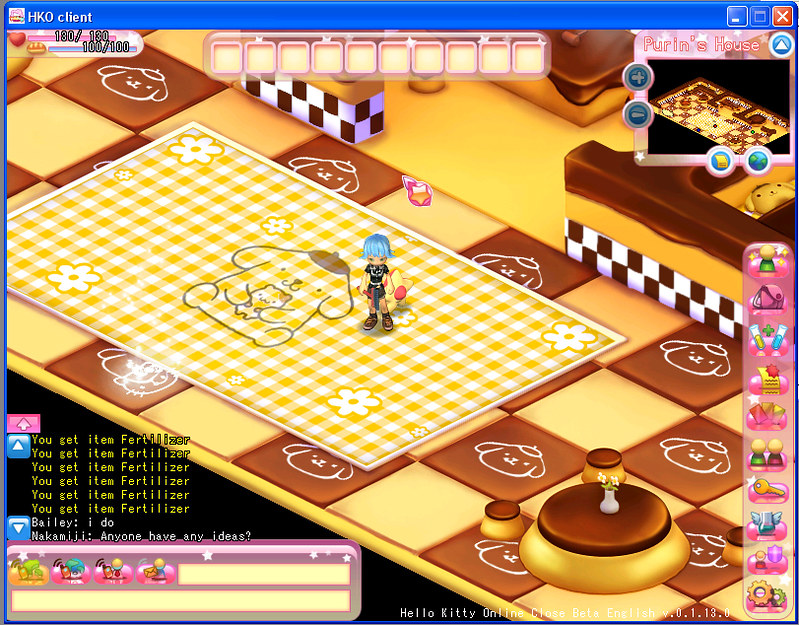This is a horizontal rectangular image, likely a screen capture of an online browser-based video game, identified as "HKO client" at the top in white text on a blue navigation bar. The central area of the image features a human avatar with blue hair, dressed in a punk rocker style, standing on a white and mustard-colored checked pad. This pad includes detailed elements such as white flowers and a brown cartoon illustration of a dog holding a smaller animal, possibly a cat. This is superimposed on a larger yellow and brown checkerboard game board, with each brown square displaying the same dog wearing a beanie. To the upper left of the main game area, there are additional game elements, including black and white squares and yellow cards, suggesting interactive components. On the right side, a series of pink squares adds more color to the scene. In the lower left, white text indicates "Hello Kitty online," and the upper right corner of the image features pink text reading "Purin's house."